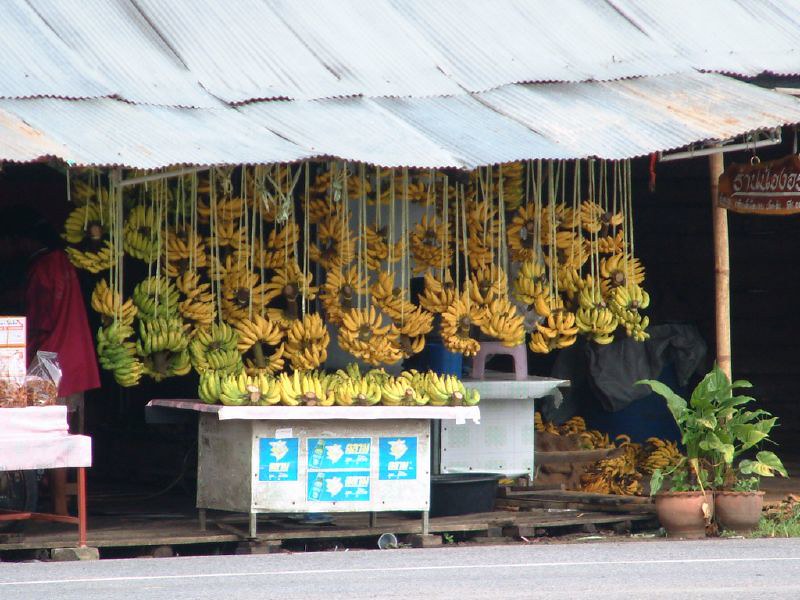In this vivid outdoor photograph of a bustling street market likely situated in a foreign country, the primary focus is a banana stand brimming with an abundance of bananas. The scene is set under a slanted corrugated metal roof, which features a partially visible sign written in an unknown foreign language. 

Hanging from the metal roof are numerous white strings suspending bunches of greenish bananas, numbering in the hundreds. Below, a sturdy gray metal table with a white top displays a selection of yellow bananas, ready for immediate sale. Adorning the front of this table are three indistinct blue signs that add a touch of color to the scene. 

To the right, gray potted plants with lush green shrubbery provide a natural border. The ground beneath is a mix of wooden pallets and gray asphalt, with scattered green grass making a subtle appearance. In the backdrop, there’s a hint of another vendor's stand, where plastic bags filled with indeterminate items and some boxes are visible along with what could possibly be either blankets or a person. A notable overstock of bananas is casually strewn on the ground, adding to the vibrant and busy atmosphere of this market snapshot.